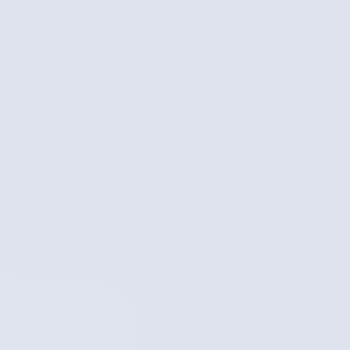The image depicts a completely blank canvas with a light gray background, resembling the color of a soft, overcast sky. The entire frame is uniformly filled with this light gray shade, with no discernible patterns, text, or illustrations. The absence of any visual elements suggests either an error in loading the image or an intentional minimalistic design. The overall effect is a serene, monochrome square that offers no further details or distractions.